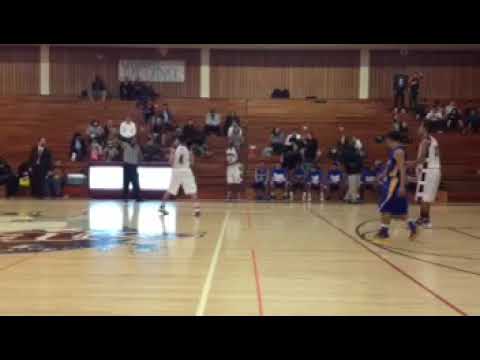The image depicts a somewhat blurry scene of an indoor basketball game, possibly a practice session, taking place on a light blonde wooden court. Two teams are present: one in navy blue or dark royal blue jerseys, and the other in white jerseys. The players appear to be standing or walking, possibly after a game reset, alongside a referee at one end of the court. The venue is an old-fashioned gymnasium with wooden bleachers, where a sparse audience, perhaps parents, is seated, implying that the event isn't highly attended. At the far end of the auditorium, behind the basketball court, there's a bright white screen. An emblem is visible on the court near the free throw line, though it's indistinct due to the image's blur.